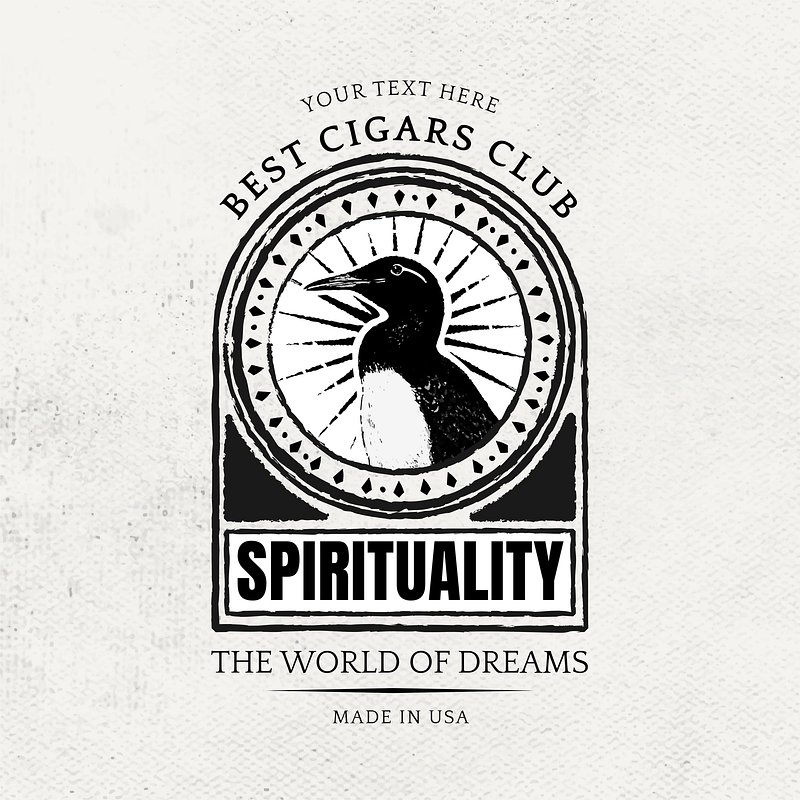The image depicts a textured white piece of paper, potentially a napkin, with an intricate black-and-white illustration imprinted on it. At the top, the words “Your Text Here” are elegantly inscribed, followed by “Best Cigars Club.” Dominating the center is a prominent emblem featuring a penguin with a white belly, facing left, and radiating a pattern of black starburst-like spikes. This central circle is adorned with concentric circular borders embellished with alternating diamonds and dots, reminiscent of the ornate designs of a vintage clock. Beneath this, in bold black lettering, the word “Spirituality” is enclosed within a rectangle, flanked by two black triangles at the bottom of the circle. Further down, the inscription “The World of Dreams” stretches across the paper, followed by a dividing line, and the phrase “Made in USA” at the very bottom. The entire layout is monochromatic, exuding a classic and sophisticated aesthetic.